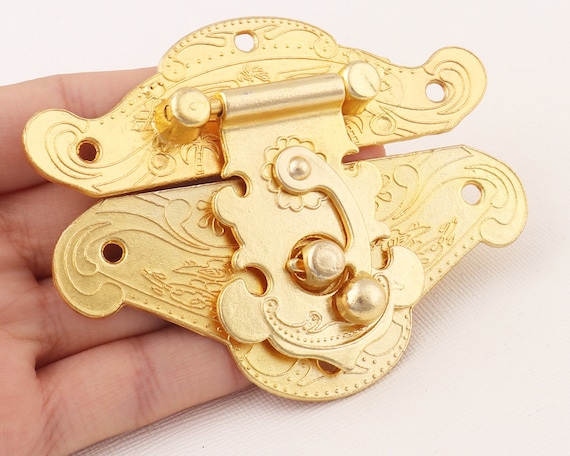In this image, a pale, off-white to light pink background sets a soft ambiance, while a hand enters from the left side, fingers holding a gold, ornate lock or latch. The hand features four visible fingers, with the thumb not in sight. The lock, intricately carved and gold-toned, features a hinged design with two distinct pieces. The upper part exhibits three prominent holes and a hook mechanism that inserts into a knob, indicative of its function to secure doors, cabinets, or gates. The object lies across the fingers, facing the camera, suggesting it is yet to be mounted. The scene is likely photographed indoors, though the time of day remains uncertain.